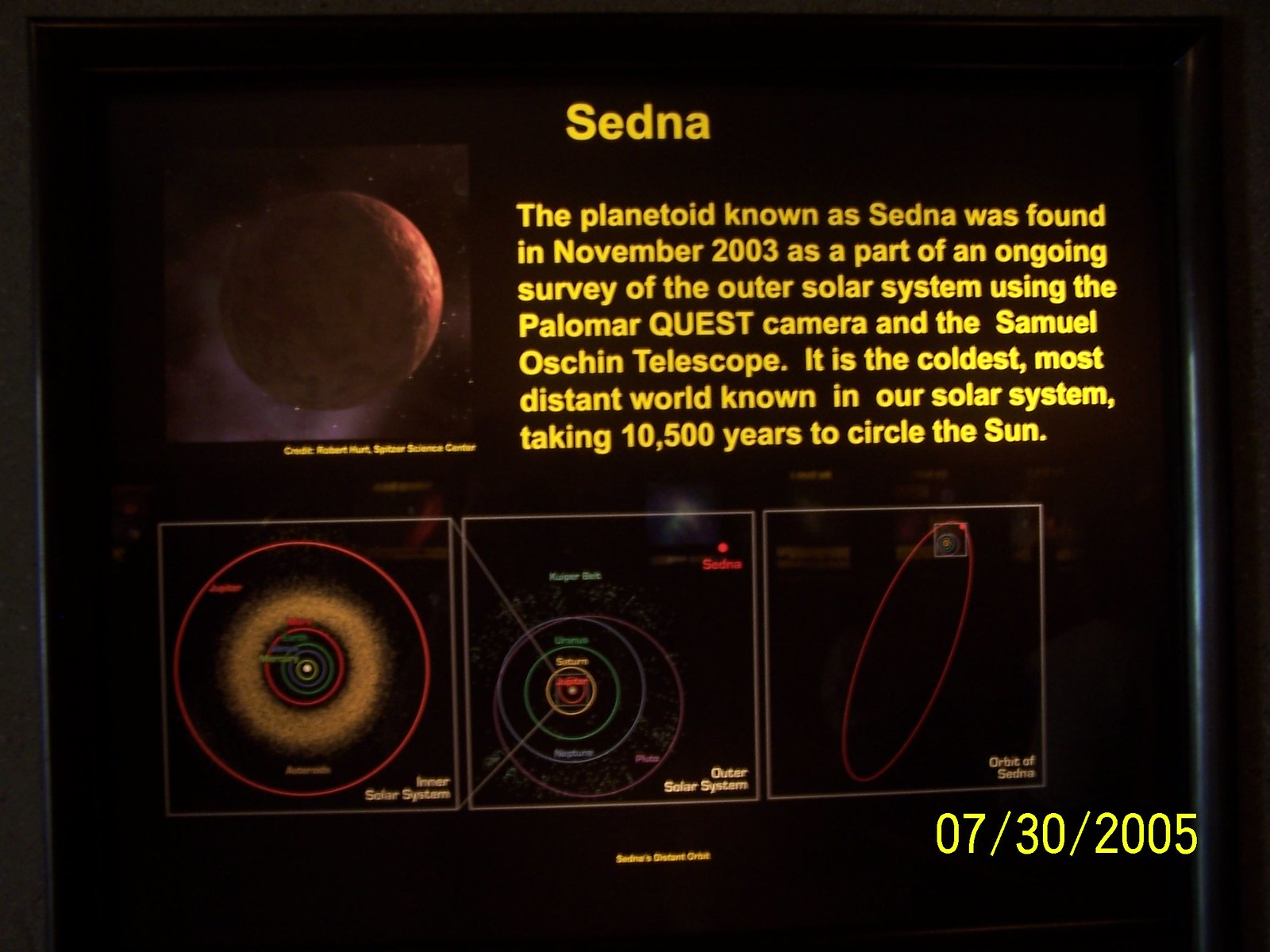This photograph, taken on July 30, 2005, showcases a dark image from a planetary or astronomy museum highlighting Sedna, spelled S-E-D-N-A at the top in yellow text. The planetoid Sedna, identified in November 2003 during a survey of the outer solar system using the Palomar Quest camera and the Samuel Ocean Telescope, is depicted. It's noted for being the coldest and most distant world in our solar system with an orbital period of 10,500 years. To the left, a picture of Sedna is visible, credited to Robert Hutt and the Spitzer Science Center beneath it. Additionally, the display includes several images illustrating Sedna's orbit within the solar system, labeled with distances from various points in the solar system.